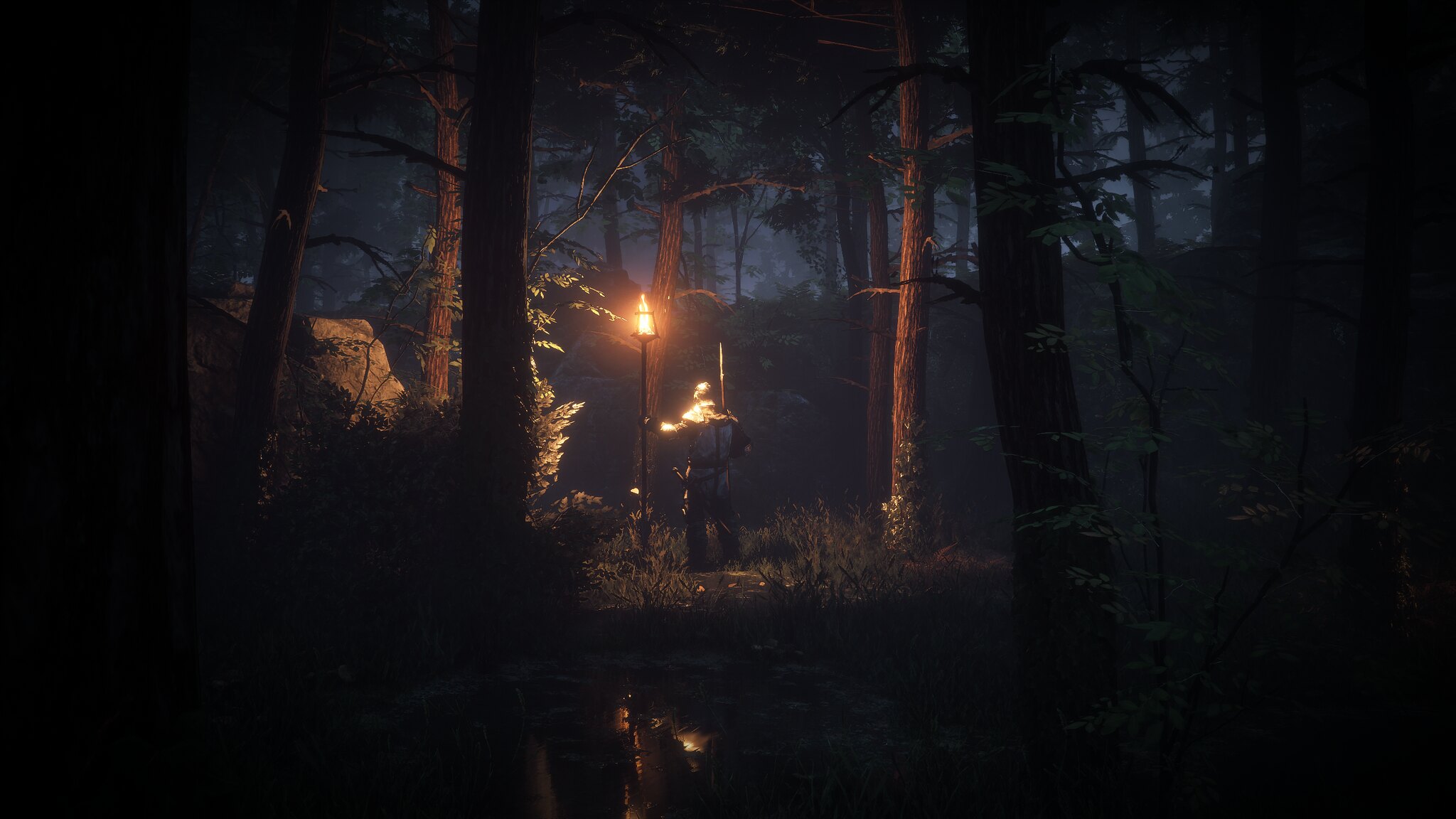This captivating image depicts a shadowy forest setting, which appears almost surreal, teetering between the realms of reality and a video game’s art. The scene is enveloped in profound darkness, with the bottom of the image entirely black, giving an impression of a mysterious void. Rising out of this inky blackness, dark trees loom in the background, their forms ghostly and indistinct. Amidst this obscurity, a figure emerges, barely visible, holding a light-topped staff. The illuminated staff casts a warm glow, revealing the rich brown hues of the encircling tree trunks and the vibrant green grass at their bases. Patches of blue sky peek through the dense canopy above, adding a contrasting splash of color to the shadowy scene. To the left, a prominent large rock stands as a silent sentinel. Below, in the blackness at the very bottom of the image, the staff's light casts a faint reflection. Besides the staff, the person appears to be wielding a spear, adding an element of intrigue and potential adventure to the scene.